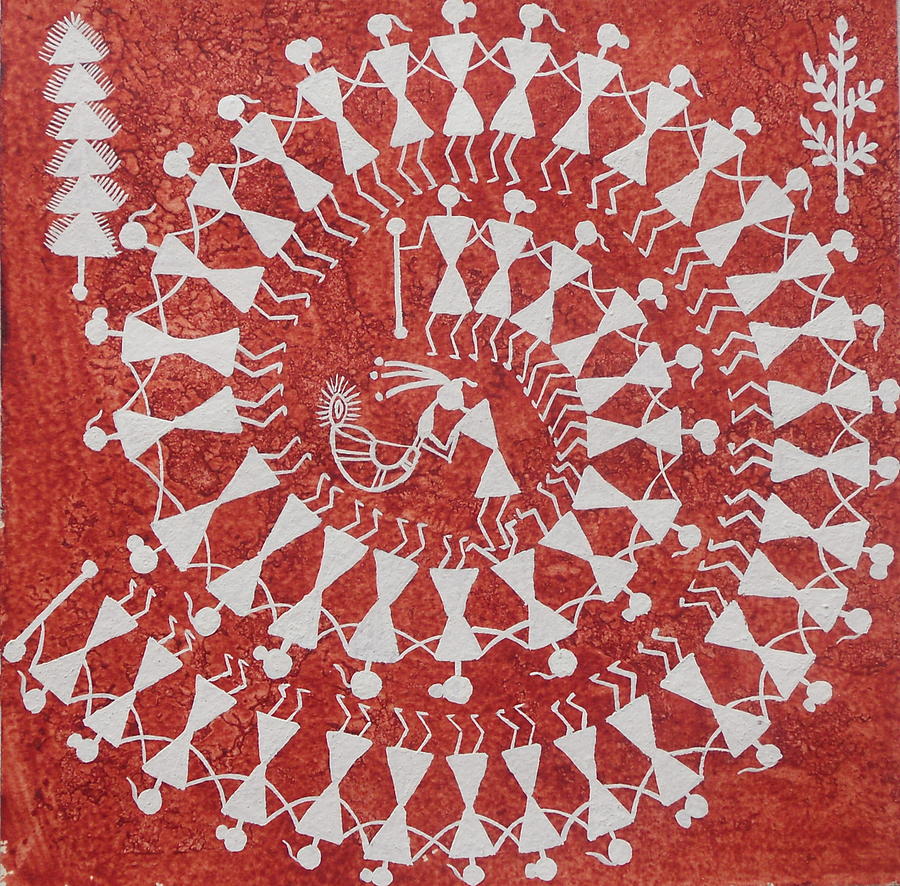Illustration Description:
This captivating red and white illustration features an indigenous art style that exudes a rich cultural atmosphere. The background is filled with a deep red hue, against which a dynamic spiral is depicted. This spiral is composed of numerous silhouetted human figures that weave gracefully from the bottom left corner of the image, coiling inward towards the center. Anchoring the center of the spiral is a prominent figure facing left, passionately blowing a large horn, which adds a sense of movement and sound to the visual narrative.

In the upper left corner of the illustration, a stylized tree is defined by six stacked triangles, evoking the geometric simplicity of a pine tree. Meanwhile, the upper right corner is adorned with a smaller, more traditionally drawn tree, adding a touch of natural diversity to the scene. The overall effect of this composition, devoid of any text, is both striking and evocative, inviting viewers to immerse themselves in its intricate details and cultural resonance.